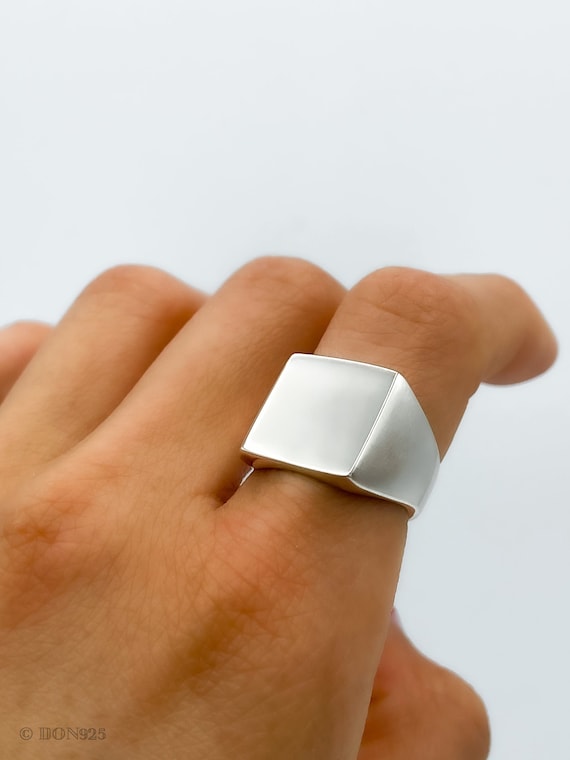This close-up photograph features a left hand, positioned with all fingers visible except the pinky finger, curving out from the lower left-hand corner. The hand belongs to a person of Caucasian descent and exhibits detailed lines in the skin. The index finger bears a tight-fitting, shiny silver ring with a thick band, which narrows underneath the finger into a somewhat triangular shape. The ring’s flat, square top, approximately one inch by one inch and lacking any gemstone, imparts a minimalist and futuristic aesthetic. The background of the image is a plain, light gray color. An inscription in the lower left corner reads "© D.O.N 925," indicating a subtle hallmark or branding.